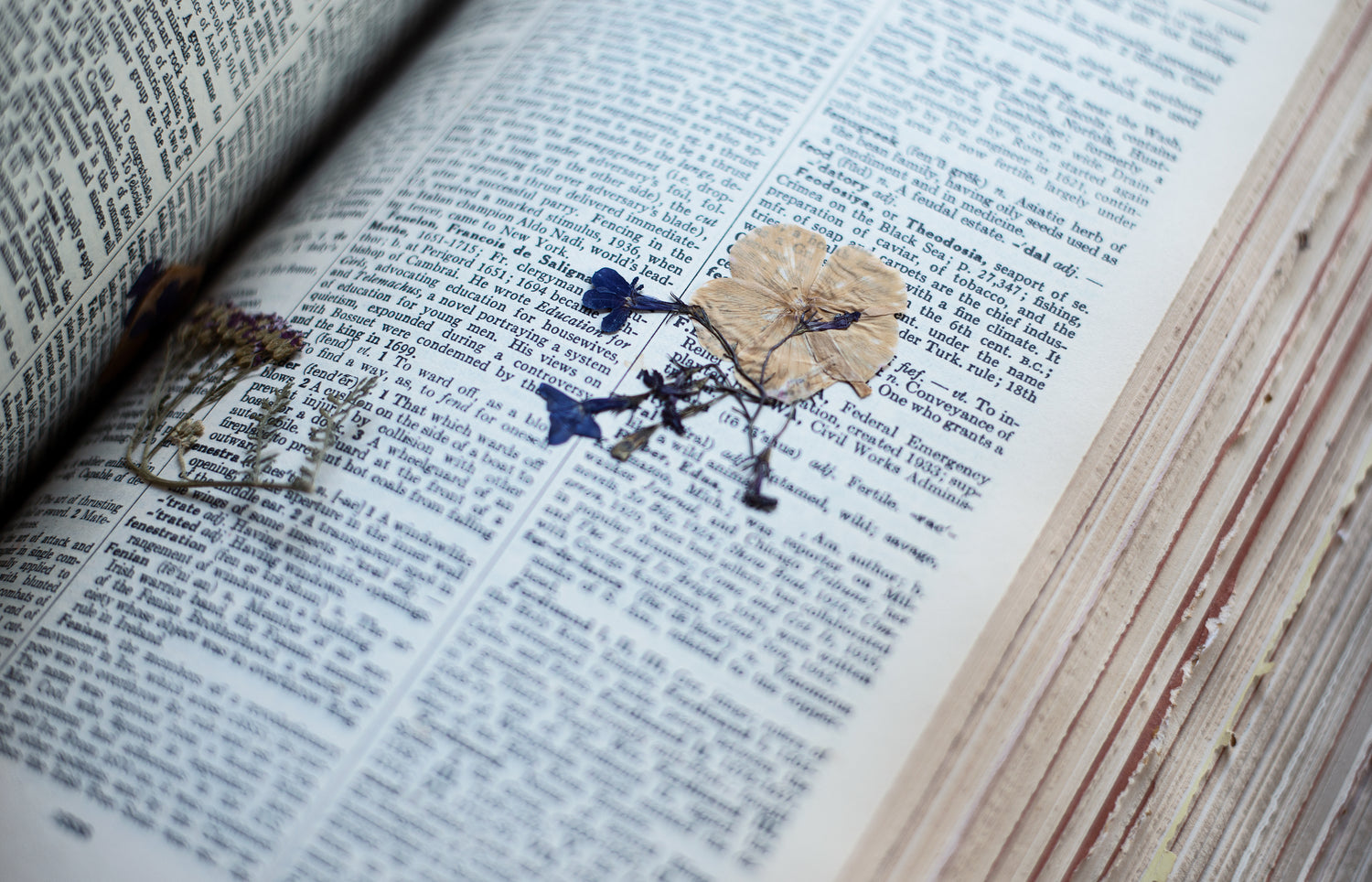This image showcases the interior of what appears to be a thick, possibly religious book, like a Bible, with white pages filled with text in a font that might be black or blue. The book is open to display two pages, with sections of the text blurred due to the tilt-shift focus of the lens, drawing attention to the pressed flowers in the center. 

Prominently featured are a cream-colored flower, potentially a tan one with green stems, centrally located and thoroughly flattened, alongside other purple-blue flowers. Closer to the book's spine, another flower with an evident purple hue is visible, accompanied by green stems that have similarly been pressed. Additionally, a yellow flower is partially stuck to the pages on the right side, contributing to the intricate, delicate nature of the scene captured in this photograph.